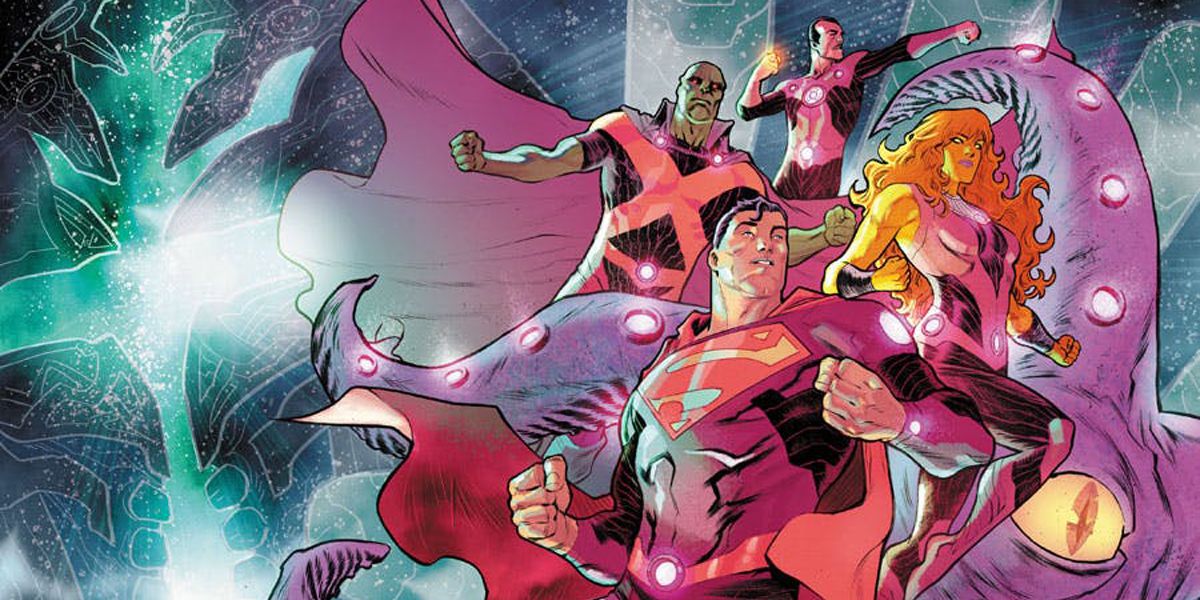In this vividly detailed comic book scene set against a cosmic background of swirling blue and green hues, four distinguished superheroes stand poised for battle. Dominating the foreground is Superman, although his traditional blue and red attire has been cast in shades of purple, possibly due to dramatic lighting. His powerful stance, with chest forward and head turned to the right, exudes readiness and determination. To his left is a striking female superhero with flowing orange hair, clad in a tight purple uniform, conveying both grace and strength. Beside her, a muscular man brandishes a bold pink letter "X" across his purple suit, exuding a sense of enigmatic power. Behind them, a male figure with a mustache and black hair, dressed in a distinct pink and brown costume, gazes into the distance, fiery power emanating from his hand. Together, they confront a formidable threat—a colossal tentacled creature lurking in the background, its presence marked by a menacing yellow eye in the bottom right corner of the image. This dynamic scene, framed by the cosmic expanse, resembles a striking poster, capturing the superheroes in dynamic poses as they prepare to face their otherworldly adversary.